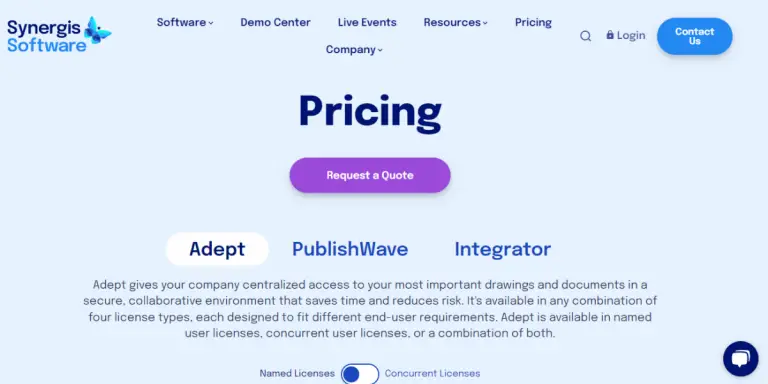The image features a long horizontal rectangle with a very light blue background. In the top left corner, "Synergist Software" is displayed, with "Synergist" in dark blue and "Software" in a lighter blue. To the right of the text, there's a butterfly with a gradient transitioning from light blue to dark blue. 

At the top center of the image, there are five tabs: "Software" (in dark blue font), "Demo Center," "Live Events," "Resources" (with a dropdown arrow), and "Pricing." Below these tabs, another dropdown menu labeled "Company" is visible. In the top right corner, there's a "Login" option, and next to it, a rounded rectangle button labeled "Contact Us."

In the center of the page, the word "Pricing" is prominent, with a purple "Request Quote" button underneath it. Beneath this section, there are three tabs labeled "Adept," "Publish Wave," and "Integrator." The "Adept" tab is currently selected, revealing detailed text below:

"Adept gives your company centralized access to your most important drawings and documents in a secure, collaborative environment that saves time and reduces risk. It's available in any combination of four license types, each designed to fit different end user requirements. Adept is available in named user licenses, concurrent user licenses, or a combination of both."

This detailed caption provides a comprehensive description of the image, capturing all visible elements and their arrangements.